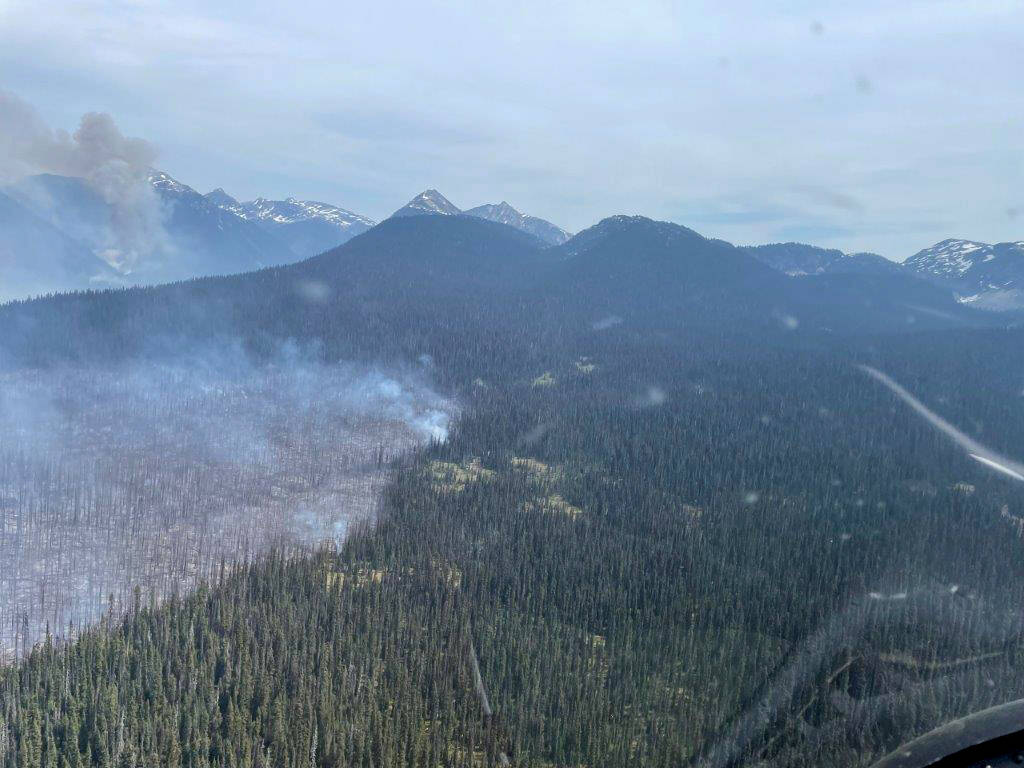This photograph, taken from a high vantage point, captures a foggy, expansive mountain range with a large forest in the foreground. The sky is a light blue with patches of gray, indicating a cloudy atmosphere. In the bottom right corner, there's a faint reflection suggesting the photo was taken through a window, possibly from a helicopter. The mountainous landscape features snow-capped peaks, particularly noticeable in the far background. On the left side of the image, a significant portion of the forest is visibly burned, with white smoke still rising from the charred trees. Additional plumes of smoke can be seen further in the distance, hinting at ongoing fires. The forest below the mountains shows varying shades of green interspersed with lighter spots where the foliage is less dense.